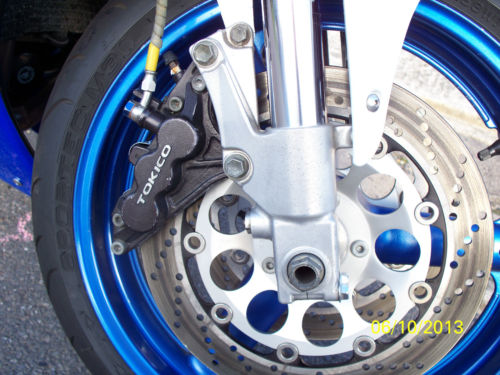This square-shaped image captures a detailed close-up of a motorcycle wheel and tire. The black rubber tire, relatively thin, encircles a bright metallic blue wheel. Prominently placed in the center is a silver hubcap with multiple circular cutouts, adding an intricate design element. Connected to this hubcap is an arm running towards the center, likely a spoke, and another metal piece that extends upwards. In the upper left-hand corner of the wheel, there's a black brake mechanism that features the name "Tokiko" in white text. A cable extends upwards from this part, probably connecting to the handbrake. The lower left corner of the image shows part of a dark gray asphalt road with a small blue object. In the bottom right corner, a yellow date mark is visible, reading "26-10-2013."